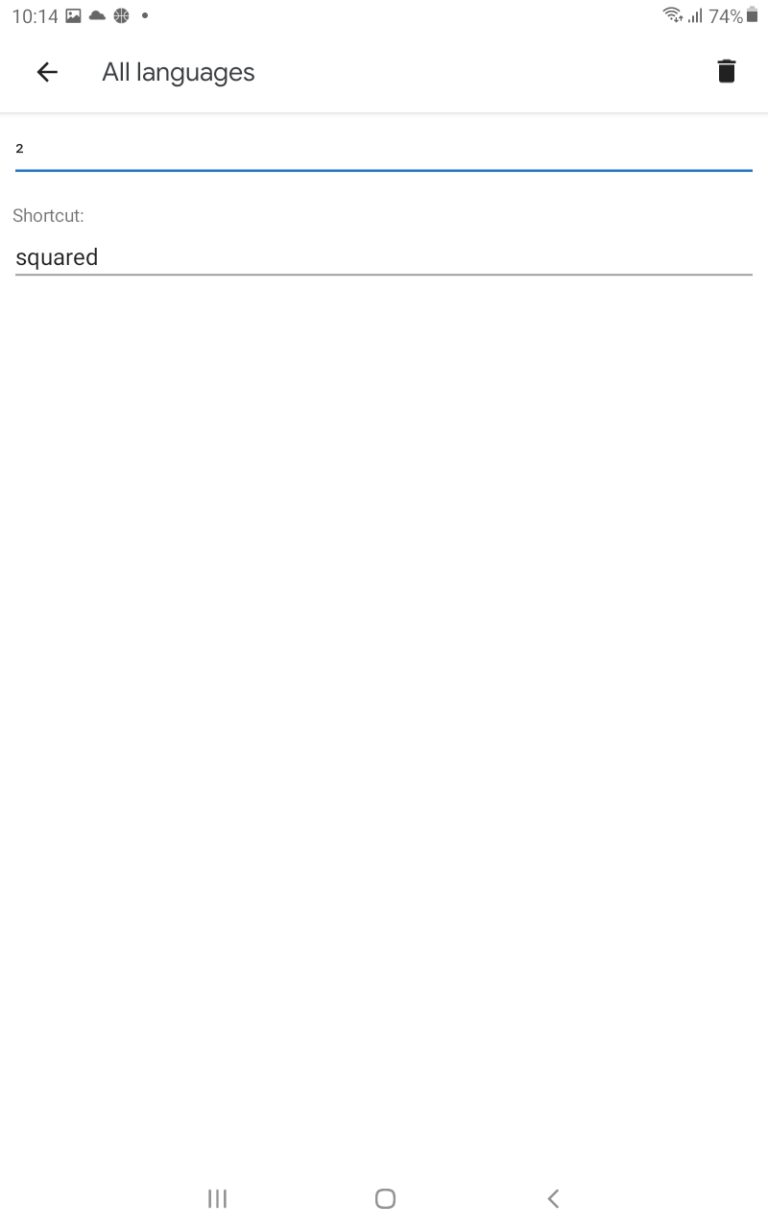The image is a screenshot of a section from an application, where various settings can be altered. At the top of the screenshot on the left, the time displayed is 10:14. On the right side of the top bar, several phone status icons are visible, including the WiFi icon, data icon, and the battery percentage, which indicates 74%. Below the top bar, on the left side, the text "All Languages" is displayed, with the number "2" directly beneath it. Below this, there is a grey header labeled "Shortcut." Inside what appears to be a text box, the word "Squared" is shown.